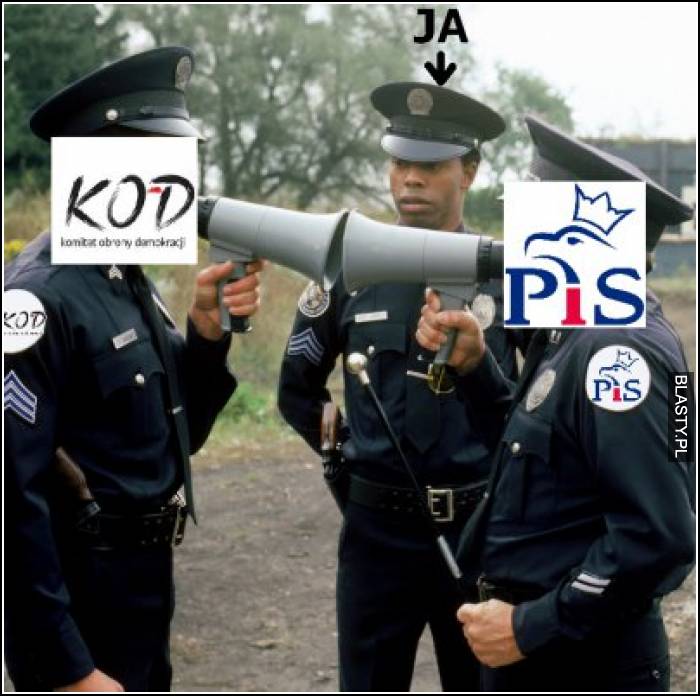In this digitally generated meme image, three police officers are standing on an unpaved road amidst an outdoor setting featuring trees, some brush, and a building to the right. The scene is in daylight with a white sky overhead. All the officers are in full uniform, adorned with badges, black ties, and hats. The two officers on the sides are facing each other, each holding a megaphone that they're using to scream at one another. The officer on the left has his face covered by a white square featuring the logo "K.O.D.," which is also seen on his shoulder. Similarly, the officer on the right has his face covered by a logo "P.I.S.," which includes an eagle with a crown and is also present on his shoulder. Both logos are in white boxes. The middle officer, who stands behind them with a perplexed expression, faces the viewer directly with "J.A." and a downward-pointing arrow above his head. He has his hands clasped behind his back. The image features colors primarily in shades of black, blue, white, green, red, and silverish hues, and the officers are positioned centrally in the frame, emphasizing the comedic and absurd nature of the meme.